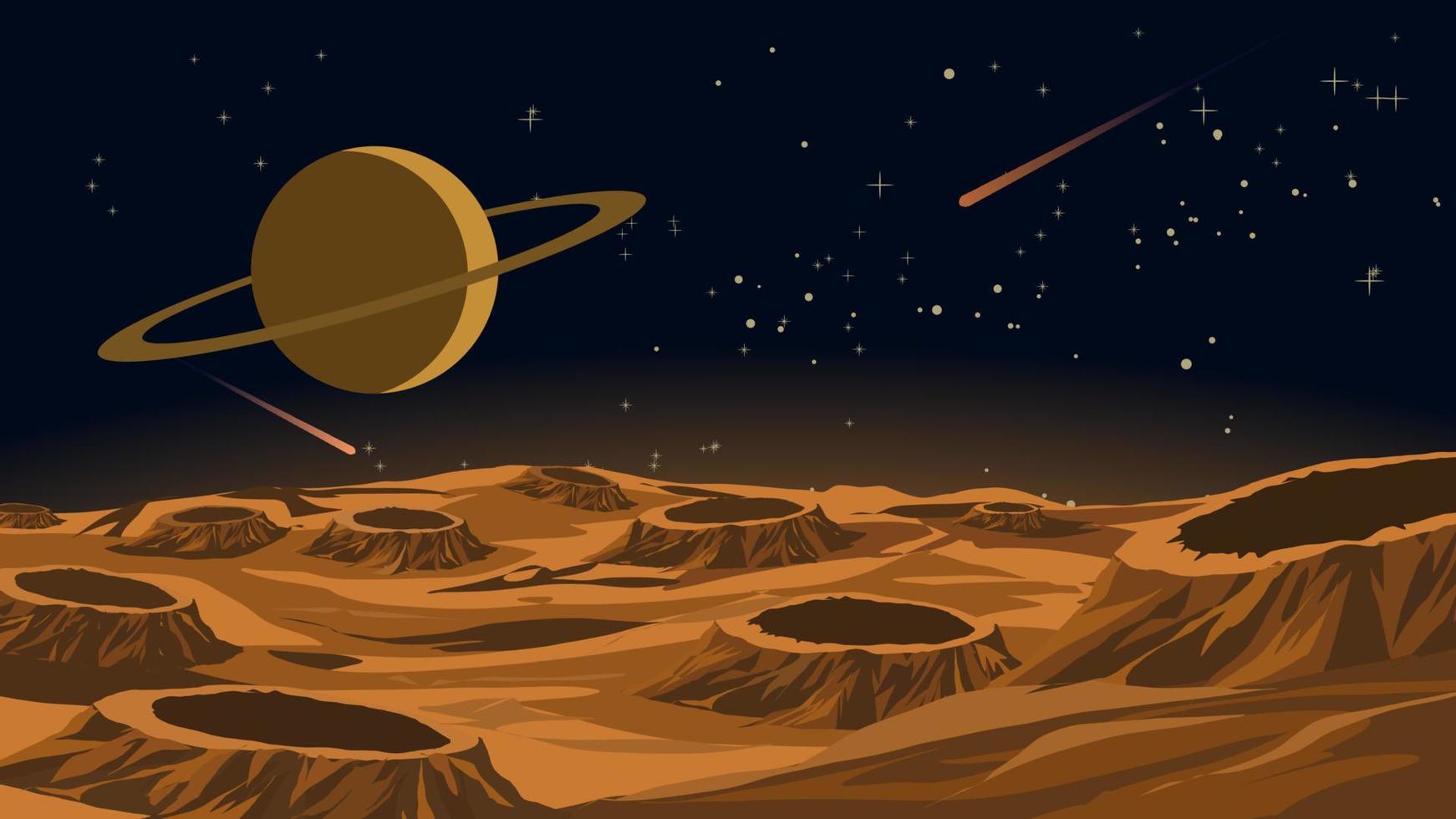This is a digital art image depicting a barren, Mars-like landscape with a rocky foreground textured in tones of browns and oranges. The surface, reminiscent of the moon, is dotted with eight distinct craters, adding a rough and cratered appearance. The land stretches across the bottom half of the image, showing an empty desert wasteland. In the background, towards the left, a tan-colored Saturn with its characteristic ring is prominently visible. The sky is filled with scattered golden stars, many rendered as little crosses or circles, and a vibrant orange shooting star streaks toward Saturn. The image, devoid of any text or individuals, captures the isolated and desolate beauty of this celestial scene.